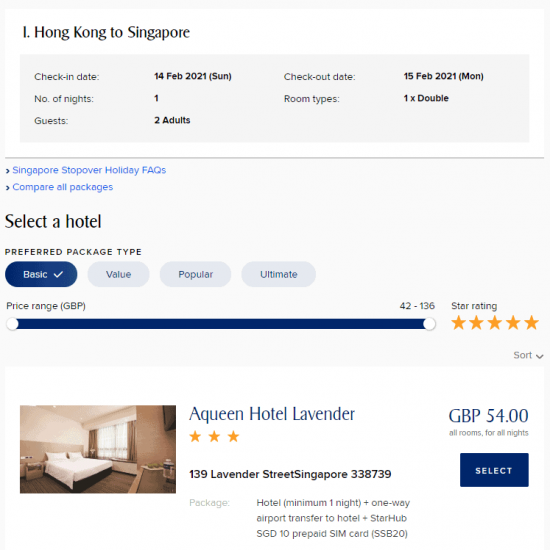Sure, here's a cleaned and detailed caption:

---

The image features a hotel booking interface. The top section displays a gray header with white text. Below this, the interface transitions to a white section with black text that reads: "Texas is one Hong Kong Singapore." Another gray text marker follows. 

Underneath this, black text states the check-in and check-out information: "Check-in date: Feb 14, 2021, Sunday. Check-out: Feb 15, 2021, Monday. Number of nights: 1. Room types: 1 Double room for 2 adults."

A gray box follows, containing text in white or blue about additional services. It lists: "Singapore Stopover Holidays FAQs, Compare All Packages, Back." 

Further down, black text prompts the user to "Select a hotel for a package type fee," followed by three buttons. The first button is blue with white text that reads: "Basic," accompanied by a check mark. The other two buttons are gray with grey text, labeled "Value," "Popular," and "Ultimate."

Next, there is a price range slider on the right, marked from 42 to 136. Below this is a star rating system showing 5 yellow stars.

The main part of the interface contains a generic hotel room photo featuring white bed linens and walls. Overlaid in bluish-purple text are the details: "Queen Hotel Lavender," a 3-star rating, and the price: "GDP 54 RGBT 54." There is also pricing information for all rooms for one night totaling "SGD 139."

Additional details include: "139 Lavender Street, Singapore, 338793."

A blue box with the word "Select" invites action. Below it, further text in black reads: "Is this premium or hotel minimum one night plus Wednesday plus one-way airport transfer fee. StarHub SGD 10 prepaid SIM: 55820."

---

This caption provides a clear, detailed description of the hotel booking interface as per the original voice input.